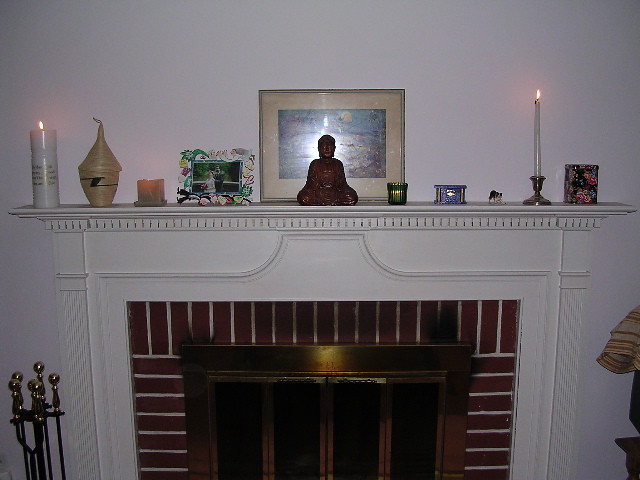This photograph captures the top two-thirds of an elegant, off-white fireplace and its mantel adorned with an array of objects. The mantel, which is white and wooden, spans most of the image, set against a matching off-white wall. Centered prominently is a brown Buddhist statue, positioned in front of a large framed painting that appears to be a softly-lit watercolor landscape.

To the left side of the mantel, a lineup of candles begins with a tall white cylindrical candle that is lit, followed by an unlit beige vase-shaped candle featuring a black 'Z'. A smaller pink candle, which appears lit despite its hidden flame, stands next to a horizontal picture frame that seems to capture a wedding photo adorned with floral designs.

On the right side of the Buddha statue, there's a small green glass candle holder containing a lit candle, a decorative blue and silver box, and a miniature figurine resembling a dog. A silver candlestick holding a tall, thin, white candle with a visible flame stands further along, followed by a decorative box in black, pink, and blue, adorned with flower patterns.

Below this meticulously arranged mantel, a red brick fireplace with a brass base and a series of black vertical rectangular windows is surrounded by brick detailing. To the left of the fireplace, a set of fireplace tools with blue ball tops and gold handles are partially visible. The fireplace itself is unlit, complementing the serene and thoughtfully decorated setting above.